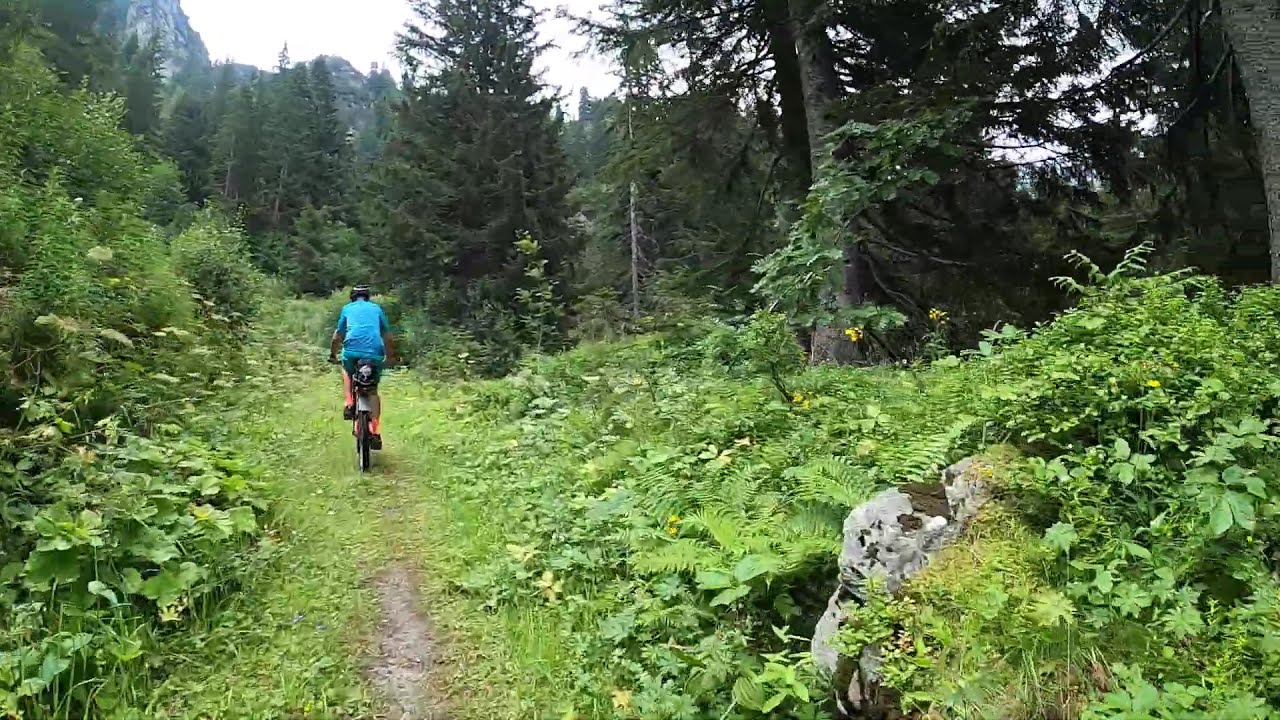The image is a detailed point of view shot capturing a narrow, overgrown countryside dirt path during the daytime. In the foreground, a person rides a black and white bicycle along the damp, grassy path, wearing orange shoes, short blue pants, a short-sleeved blue shirt, and a black helmet. The path is so narrow it only accommodates a single cyclist and is bordered by lush, dense vegetation, including various ferns and ivies. In the lower right corner, a large moss-covered boulder peeks through the greenery. Further in the distance, the path winds towards towering green pine trees, alongside a majestic cliff and mountain range, all set against a foggy grayish-white sky. The overall scene is reminiscent of a jungle or dense forest, rich with vibrant, untamed plant life.